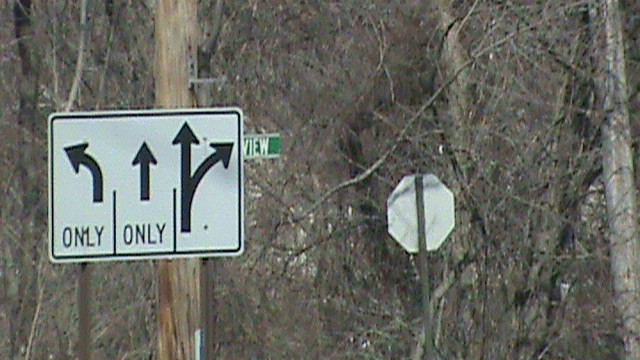The image depicts a dreary, colorless scene dominated by a dense, leafless mass of trees in drab shades of light tan, gray, black, and charcoal. On the left-hand side of the image, a rectangular white traffic sign, outlined in black, is attached to a wooden utility pole. This sign is divided into three sections, each with different directional arrows: the leftmost arrow curves left and reads "Only," the center arrow points straight ahead and also reads "Only," and the rightmost arrow points straight ahead with an additional rightward curve, indicating that the lane can either go straight or turn right. Peeking out from behind this utility pole is a green street sign, showing only the word "view" in white letters. Just right of the image's center, you can see the back of a silver stop sign facing the dense tree background.